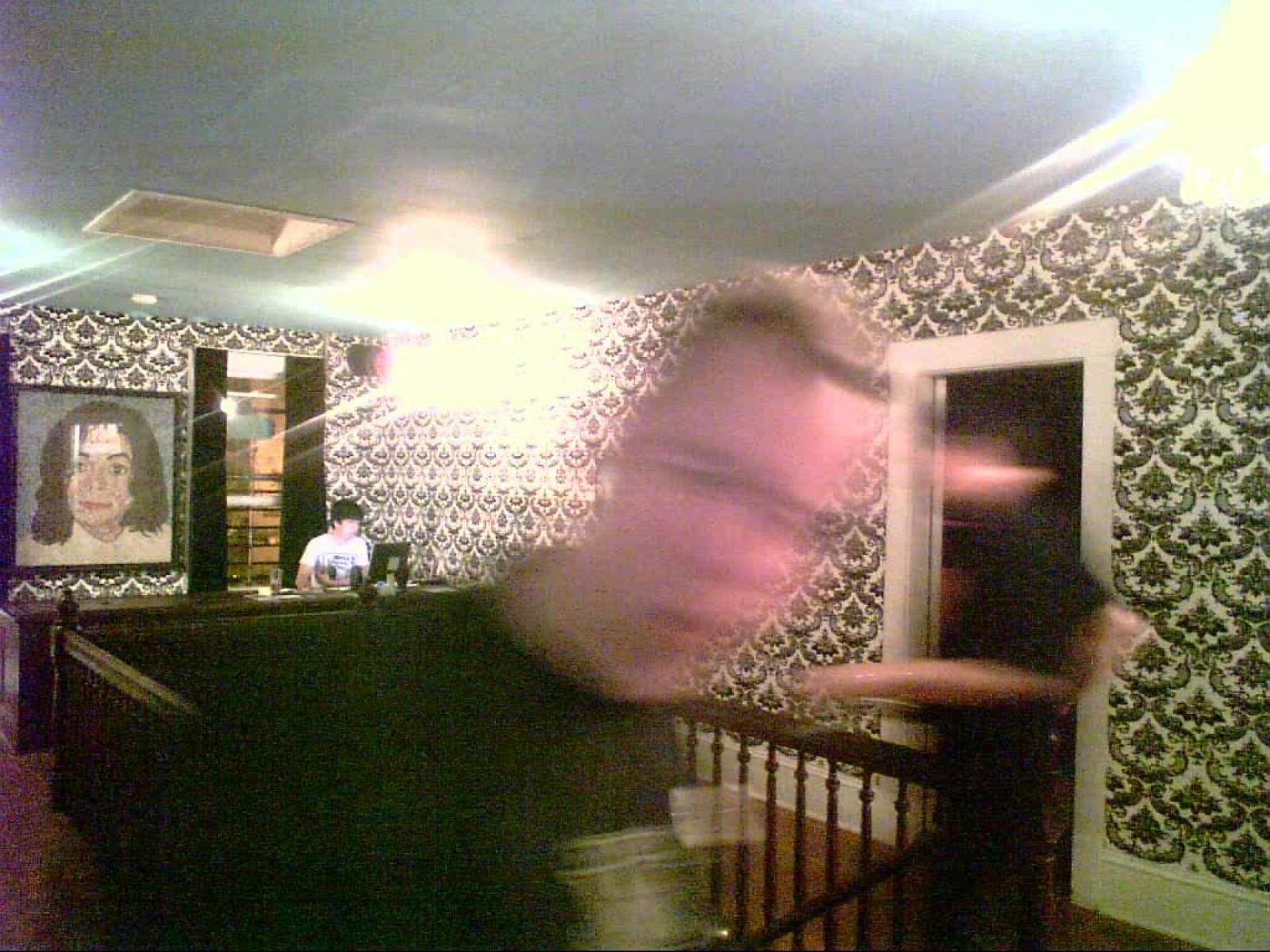The photograph features an up-close, blurry image of a man who appears to be taking a selfie. Although the subject's features are indiscernible due to the blur, you can tell that he is a white male by his haircut and general face and brow shape. He is wearing a black t-shirt. The setting appears to be an entrance area or room with a wooden stairwell descending in the background. The walls are adorned with a busy black-and-white wallpaper. In the far end of the room, another man is visible, sitting at a desk engrossed in looking at a laptop or a small monitor. A window is positioned behind him, and hanging on the wall next to him is a drawing of Michael Jackson.